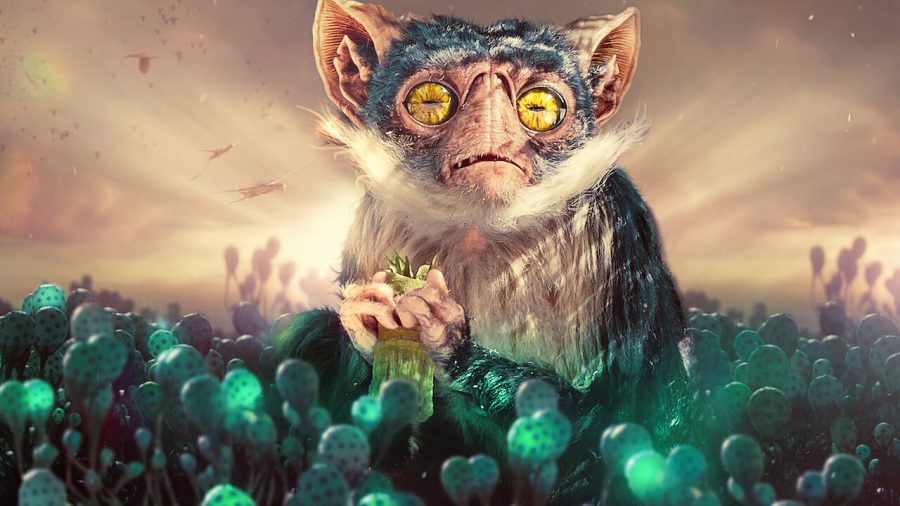The image is a detailed sci-fi fantasy depiction of a unique, large creature that resembles a hybrid between a cat, monkey, and bat. It has fur that is predominantly gray, but the face, ears, and paws are tan-colored. The creature’s notable features include enormous, round yellow eyes with unusual horizontal slits, a wispy white beard flaring towards its bat-like triangular ears, and a downturned mouth slightly ajar. The creature's hands are clasped in front of it, holding an object that appears to be a jar with greenery. It stands in a field filled with short-stemmed plants, each topped with green orbs dotted with darker green spots, resembling an alien landscape. The background features an ethereal, beige and brown sky with a sun that appears to be rising or setting, casting streaks of light and shadows across the creature's fur. There are faint clouds and indistinct flying objects in the sky, contributing to the fantastical atmosphere. The overall color palette is muted, with greens, tans, browns, grays, and blacks blending harmoniously.